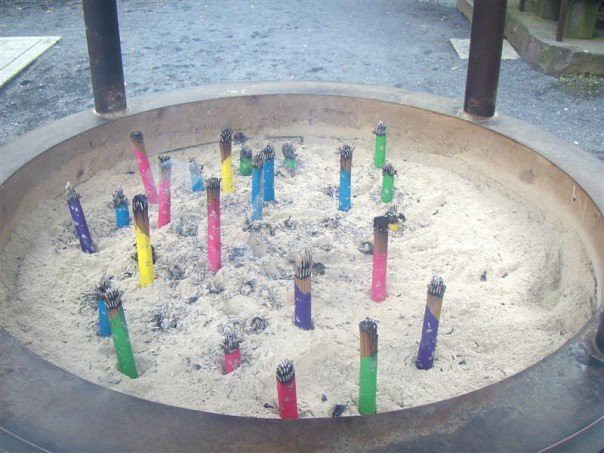The image captures an outdoor setting featuring a large, circular concrete structure filled with white sand and scattered with black ashes. Sticking up from the sand are numerous brightly colored, cylindrical objects in shades of yellow, green, pink, blue, purple, and red. These objects, which appear to be partially burned incense sticks, are singed at the top. Surrounding the structure are two metal poles, positioned at the top part of the photo. The background is a gray, gravelly area with a concrete curb in the upper right corner and a concrete tile in the upper left. The overall scene suggests a place of ritual or offering, where the burnt incense sticks create a stark contrast against the white sand and blackened remnants.